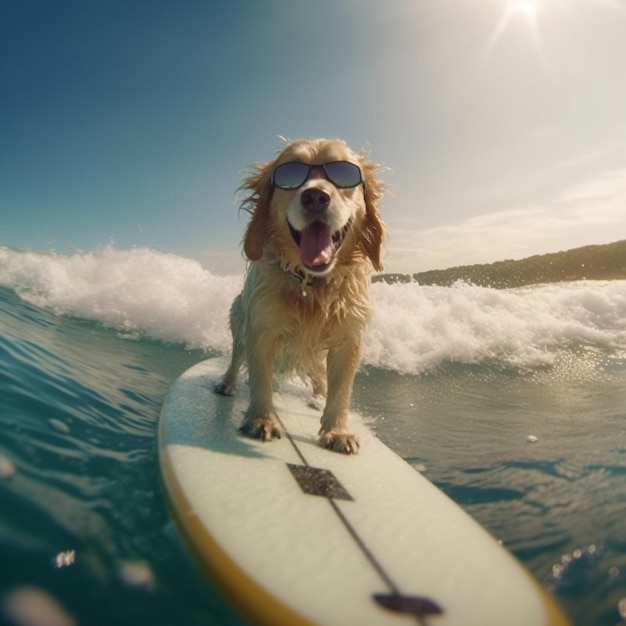This close-up photograph captures a golden retriever joyfully surfing on a white and yellow surfboard in the ocean. The dog, with its long, wet blonde hair glistening in the sunlight, wears reflective black sunglasses, giving it a cool, confident look. Its mouth is open in a wide, happy smile, tongue lolling out as it enjoys the ride. The surfboard, characterized by a black line running down the middle adorned with square and oval shapes, is pointed directly towards the camera. The wave behind the dog crests with white caps, while the blue and green water adds vibrant contrast to the scene. Water droplets are visible on the camera, highlighting the action. The sky above is a clear blue with a few clouds, and in the top right corner of the image, a distant landmass can be seen, completing this picturesque moment of canine surfing bliss.